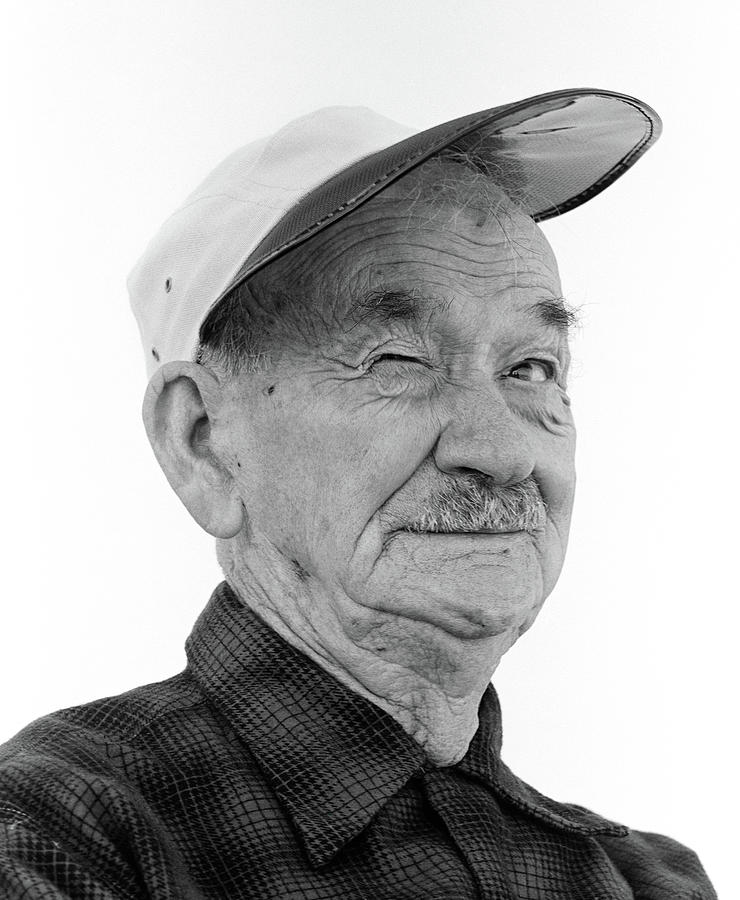This black-and-white photograph portrays an elderly man from the shoulders up, wearing a white baseball cap with a shiny, reflective dark visor. His gray mustache is neatly positioned above his upper lip. He sports a black plaid shirt, buttoned up to the top, with a distinct pattern of small squares. The man exudes a jovial aura, winking his right eye (on the left from our perspective) while looking to the left. His face, adorned with bushy eyebrows, displays numerous wrinkles, especially around his eyes and forehead, emphasizing his advanced age. His neck also shows signs of age, adding to the characteristic features of an elderly individual. Despite his apparent age and the possibility of having lost his right eye, his expression conveys a spirited and happy demeanor. The white backdrop further accentuates the details of his features and attire.